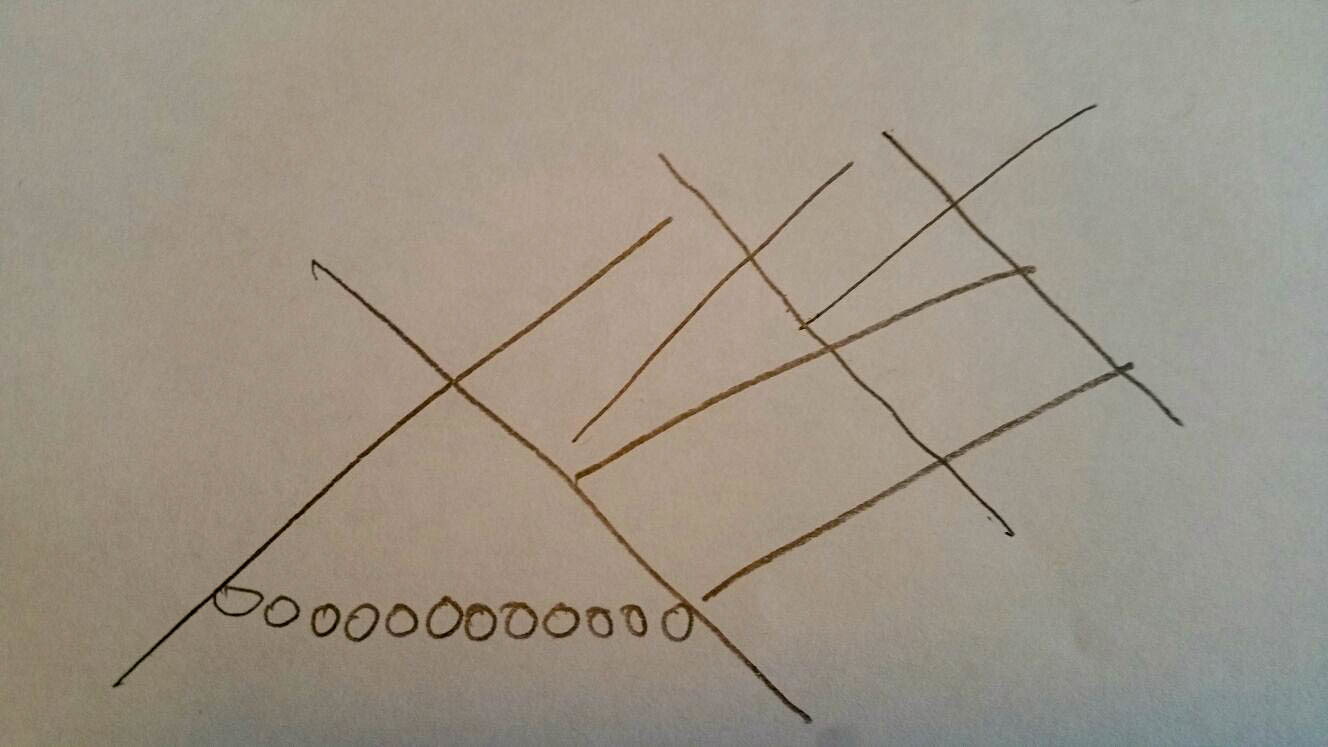The image features a meticulously drawn geometric composition on an off-white piece of paper, created using pencil. Dominating the artwork are three straight vertical lines interconnected by two horizontal lines at the lower and mid sections, forming a structural framework. Emerging from the middle vertical line, a diagonal line extends outward, intersecting the third vertical line. Above this, another diagonal line originates near the middle bar, stretching almost to the far left before crossing the third vertical line. Additionally, the far left vertical line has a diagonal line that extends almost to the middle line and then angles sharply left to form a triangular shape. Nestled within this triangle are twelve carefully placed circles, adding a layer of intricate detail to the overall geometric arrangement.